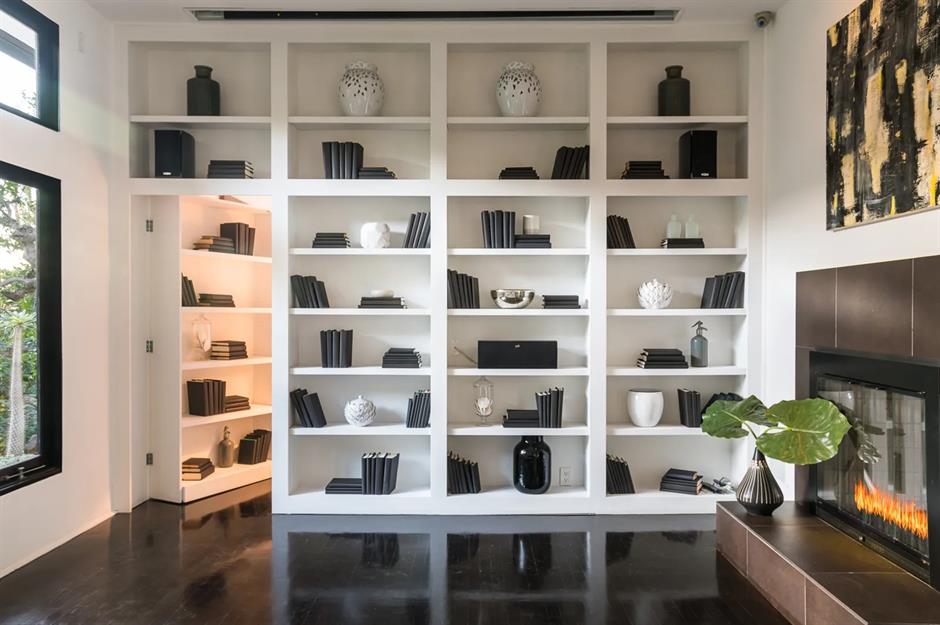The photograph depicts a meticulously organized, modern living room. The focal point is a large wall, extending from left to right, adorned with a built-in shelving unit arranged in a precise grid pattern. The top section features eight uniform, independent shelves—two rows of four shelves each—groaning with immaculately arranged, black-and-white ornamental pieces including books, vases, candles, and bowls. Below these, from the ceiling to near the floor, are four columns and five rows of smaller compartments. One of these compartments, located on the far left, cleverly doubles as a hinged door leading to a hidden room bathed in a warm orange glow.

The room maintains a monochromatic theme, where even the blackish wooden floor gleams beneath the pristine white and black decor. To the right, a sleek, LED-lit fireplace adds warmth to the setting, accompanied by a neat planter positioned beside it. Above the fireplace hangs a modern black-and-white artwork, enhancing the room’s contemporary feel. Additionally, a security camera is discreetly mounted in the upper right corner, while sunlight streaks in from partially visible windows with black frames on the left wall, providing a touch of natural light to this epitome of organized, stylish living.